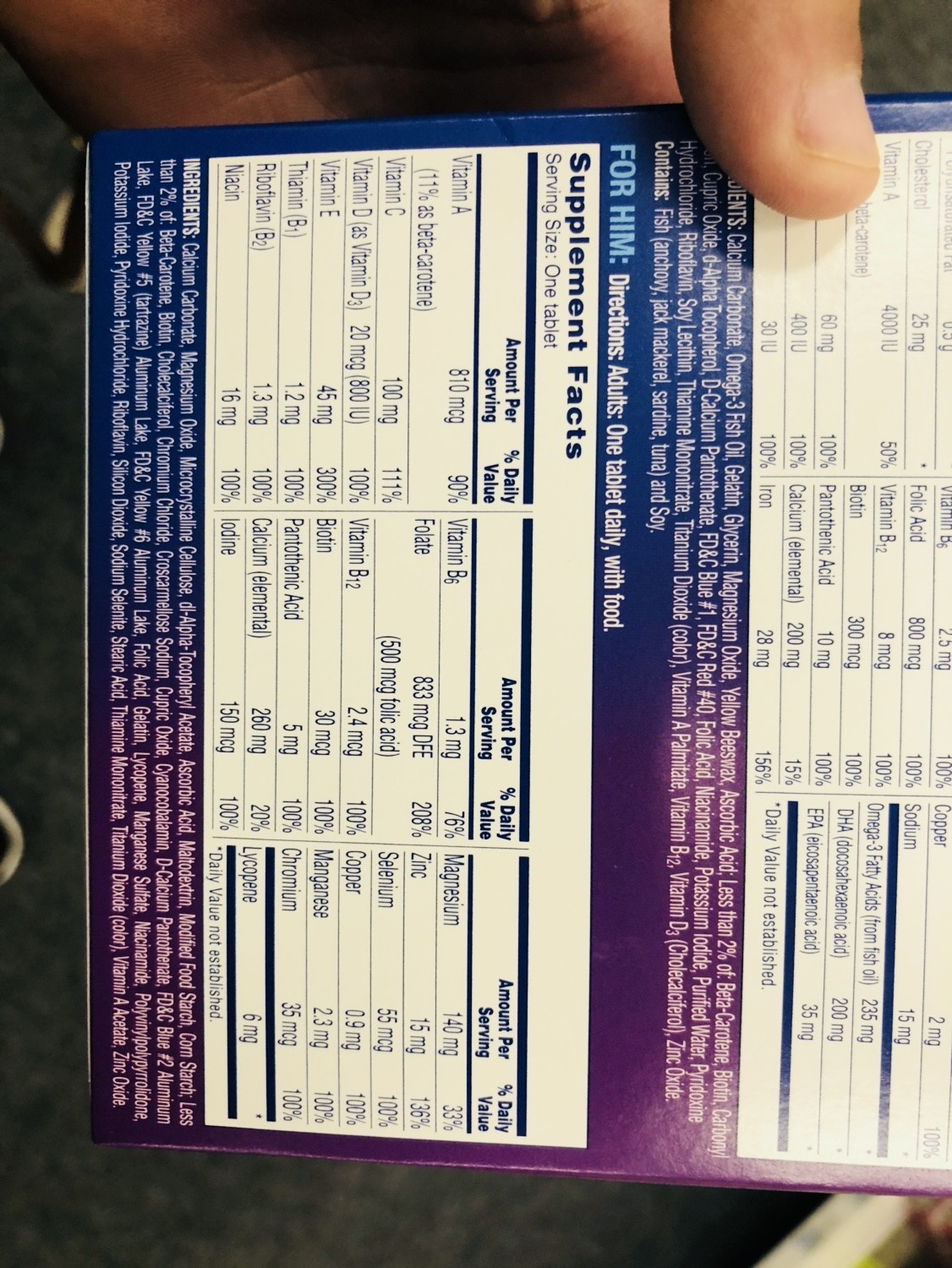This image shows the back of a rectangular, sideways-rotated purple box held by a hand with fair Caucasian skin and short nails. The box closely resembles packaging of a vitamin or supplement product. Due to the rotation, the top of the package appears on the right-hand side, and the bottom on the left. A significant portion of the visible text is dedicated to nutritional and supplemental information, primarily displayed in white lettering against a dark blue background. A highly noticeable text segment reads, "For Him, Directions: Adults, One Tablet Daily with Food," suggesting the product is a specific supplement. Supplement facts including vitamins A and B, among others, are also listed, with details on serving sizes and daily percentage values, making it clear this is not food but a dietary supplement. The background of the image is a blurry blue, and there is a thumb visible at the top of the photo, holding the box.